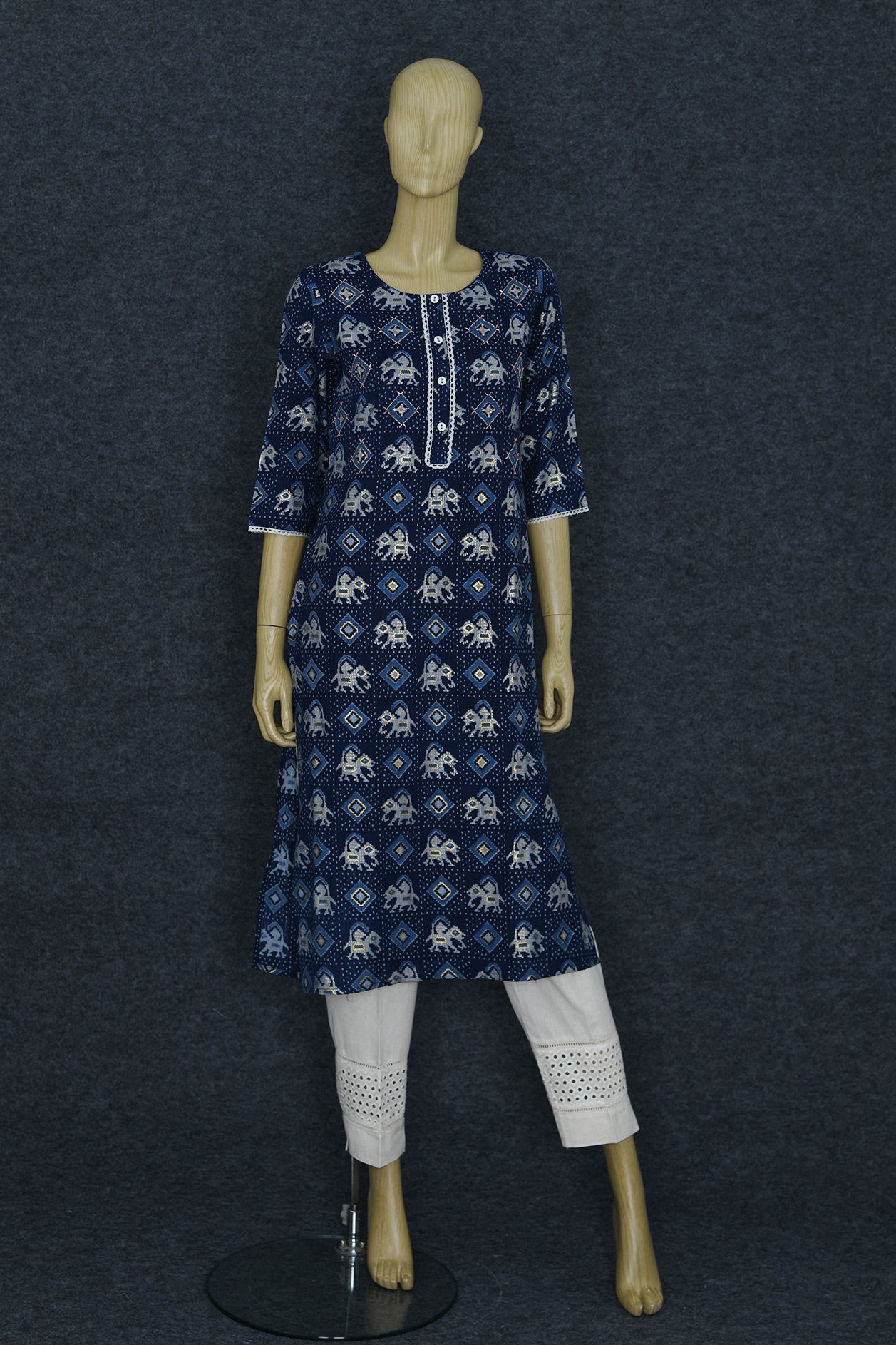This photograph features a tan, bald female mannequin with an unpainted, blank face, positioned against a denim blue background. The mannequin is secured on a pedestal by a metal stand that runs up its right leg, which is attached to a black disc at the base. She is dressed in a knee-length blue garment that lies somewhere between a tunic and a dress, reminiscent of attire typically worn by Indian women when not in a sari. This blue dress has a mix of darker and lighter blue shades and is decorated with intricate white patterns and features a row of four buttons down a placket in the front. Underneath the dress, she wears white, three-quarter length pants that have embroidered rings of holes around the cuffs, just above the ankles, revealing her bare feet. The mannequin's hands are also bare, contributing to the overall minimalist aesthetic.